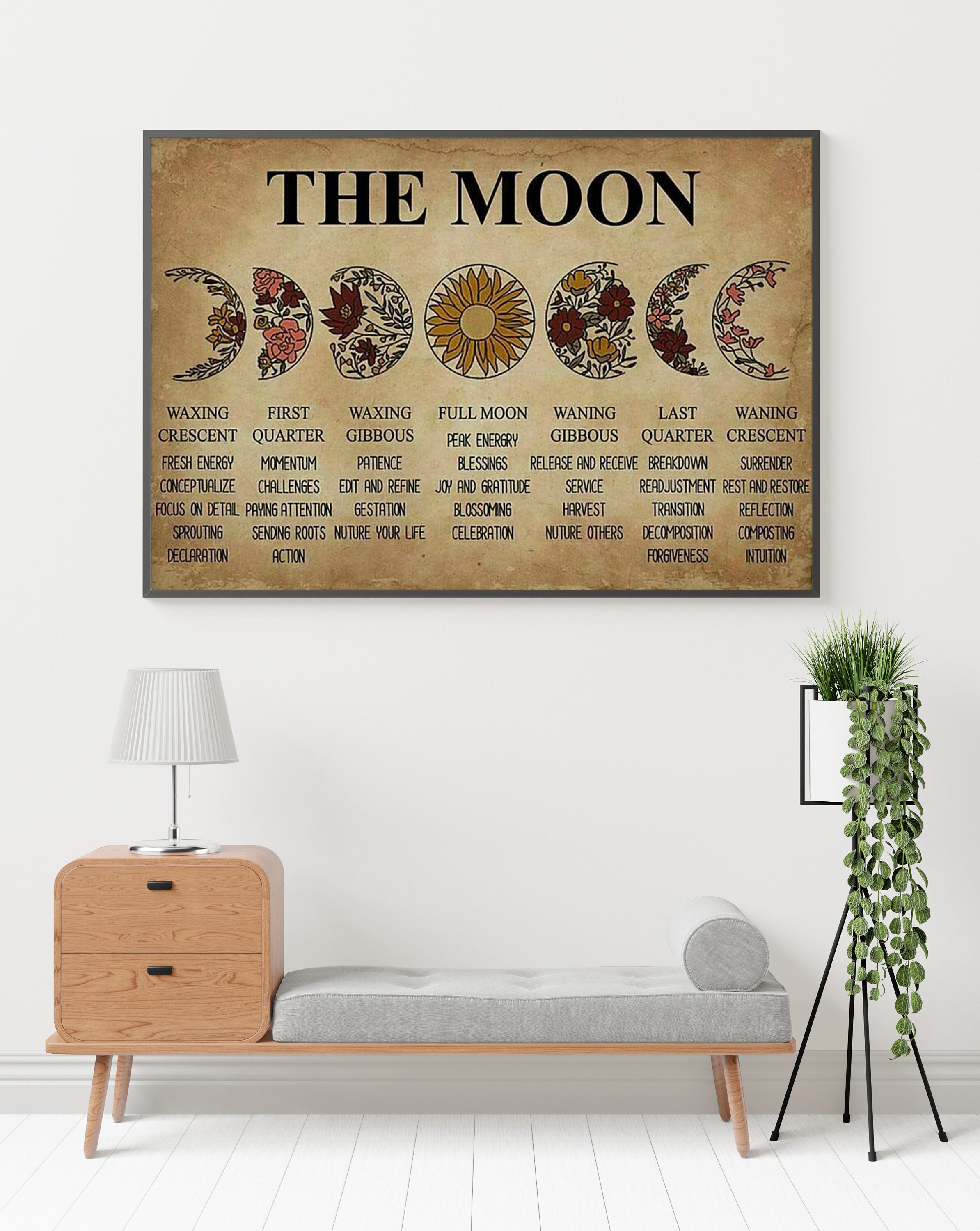The next picture in the set showcases a cozy living room corner featuring a wall-mounted illustration of the moon phases labeled with the stages: Waxing Crescent, First Quarter, Waxing Gibbous, Full Moon, Waning Gibbous, Last Quarter, and Waning Crescent. The moon illustrations appear whimsical and animated, with occasional flower motifs integrated into the design. Below the artwork, there is a small day bed with a thin gray cushion and a round gray pillow on the right. Flanking the day bed on the left are two brown drawers resembling nightstands, topped with a silver-bottom lamp with a white shade. To the right, a white cylindrical planter hosts a grass-like plant, complemented by an ivy-like plant with rounded, light gray-green leaves cascading down.